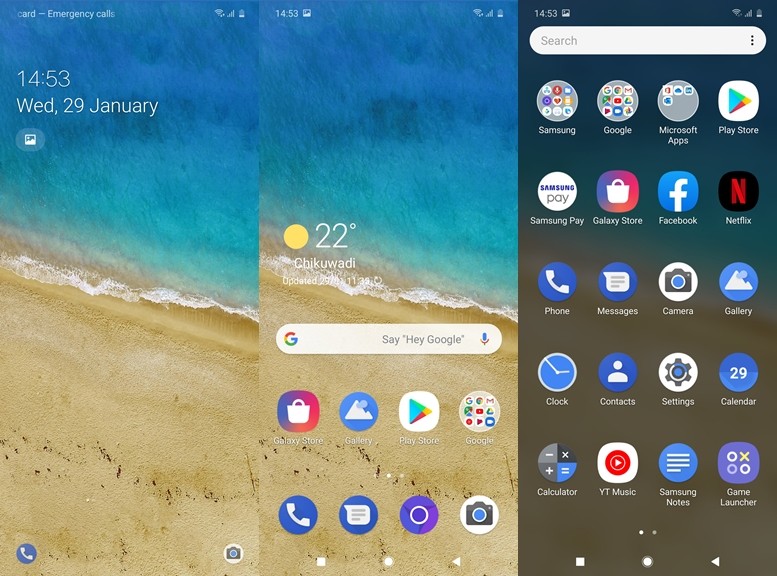Screenshot of a smartphone home screen featuring a vibrant beach-themed background with blue ocean waves and sandy shore. Displayed prominently on the top part of the screen is the date, "Wednesday, 29 January," and the time in military format, "14:53." The screen is populated with various app icons, including Samsung Pay, Gallery, Camera, Clock, Contacts, Settings, Calendar, YT Music, Samsung Notes, Game Launcher, Google Play Store, Microsoft Apps, Galaxy Store, Facebook, and Netflix. At the bottom, there is a Google search bar with the prompt, "Say 'Hey Google'.